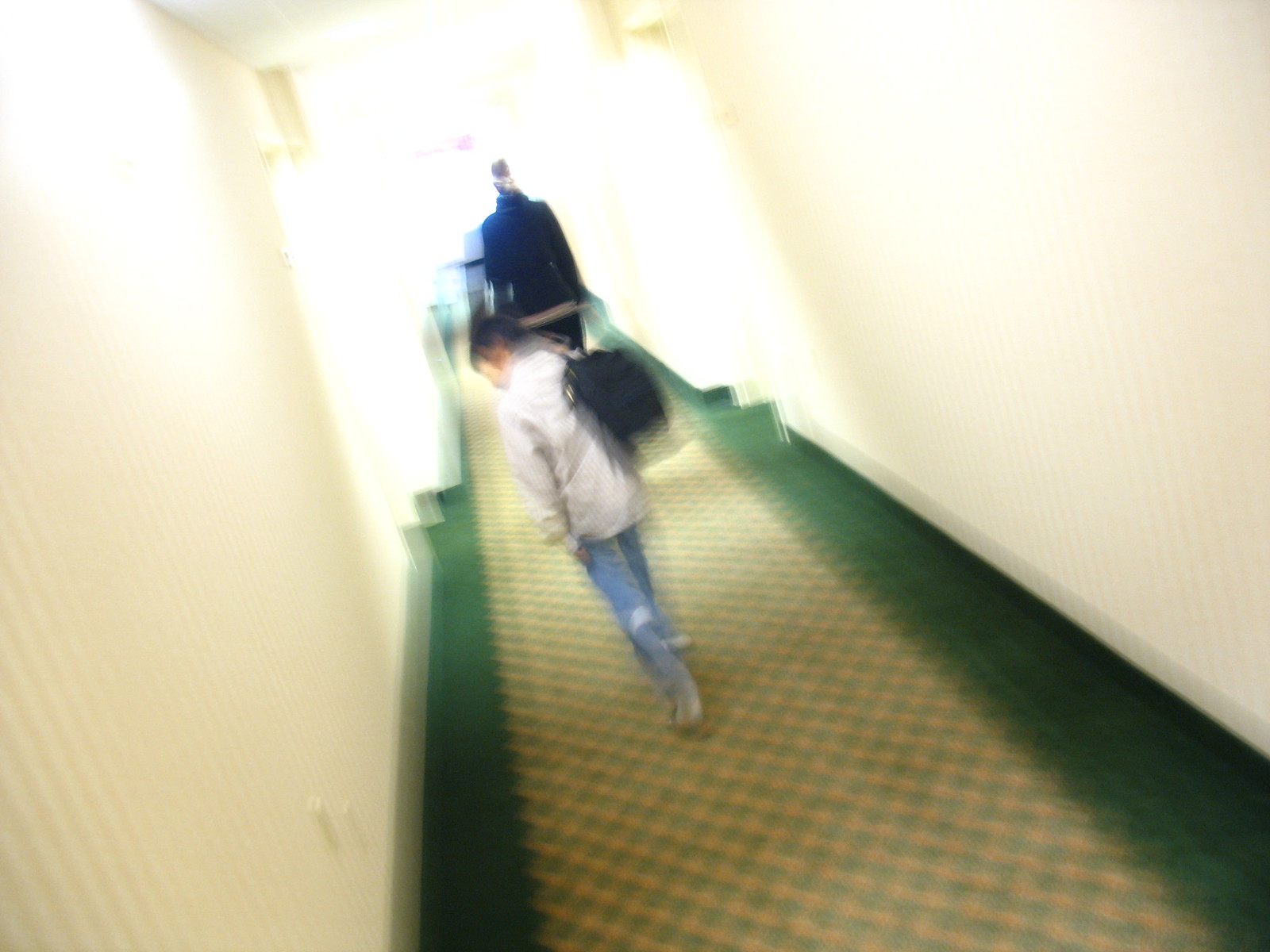This color photograph, taken from a slight angle and in landscape orientation, captures an interior carpeted hallway, possibly in a hotel or similar facility. The hall is carpeted in a distinctive pattern featuring forest green and cream-colored checks with dark green edges. The white walls of the hallway are brightly illuminated, adding to the overexposed and highly unfocused nature of the image. In the center of the photograph, a young child wearing jeans, a light-colored jacket, and a black backpack walks down the middle of the carpet, looking down. Walking ahead of the child is an adult, possibly a male, dressed in a black tracksuit-like outfit. Both figures are moving towards a glaringly bright light source at the end of the hallway, which further contributes to the image’s overexposure and blurriness. The camera's tilted angle and the overall lack of focus give the scene a dreamy, almost surreal quality.